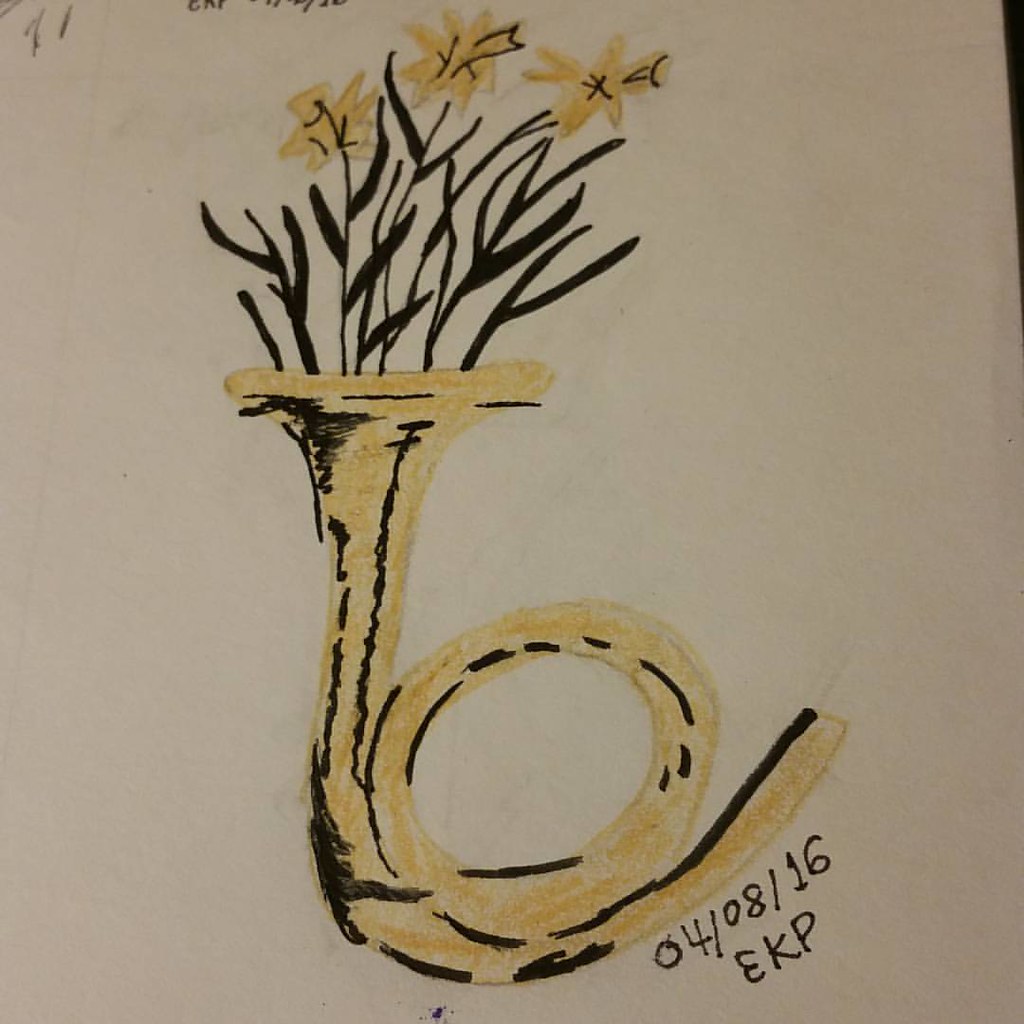The photograph captures a detailed drawing on a pristine sheet of white paper. The focal point of the artwork is a meticulously sketched brass horn or trumpet, which elegantly loops into a circular shape. The instrument, predominantly gold-colored, features intricately shaded black areas to represent shadows, enhancing its three-dimensional appearance. The drawing's precision extends to the mouthpiece at one end and the flaring bell at the other.

Beneath the mouthpiece, the artist has inscribed "04-08-16 EKP," indicating perhaps the date of the creation and the initials of the artist. Emanating from the bell of the horn are delicate flowers, characterized by their black stems and leaves. Three blossoms are prominently displayed, their petals boasting a striking yellow hue juxtaposed with black highlights, adding depth and contrast to the composition.

Above the main drawing, at the very top edge of the image, there is additional text. However, this writing is partially cut off and illegible, leaving a hint of mystery about what further information it might convey. This thoughtful and symbolic integration of musical and natural elements makes for a captivating visual experience.